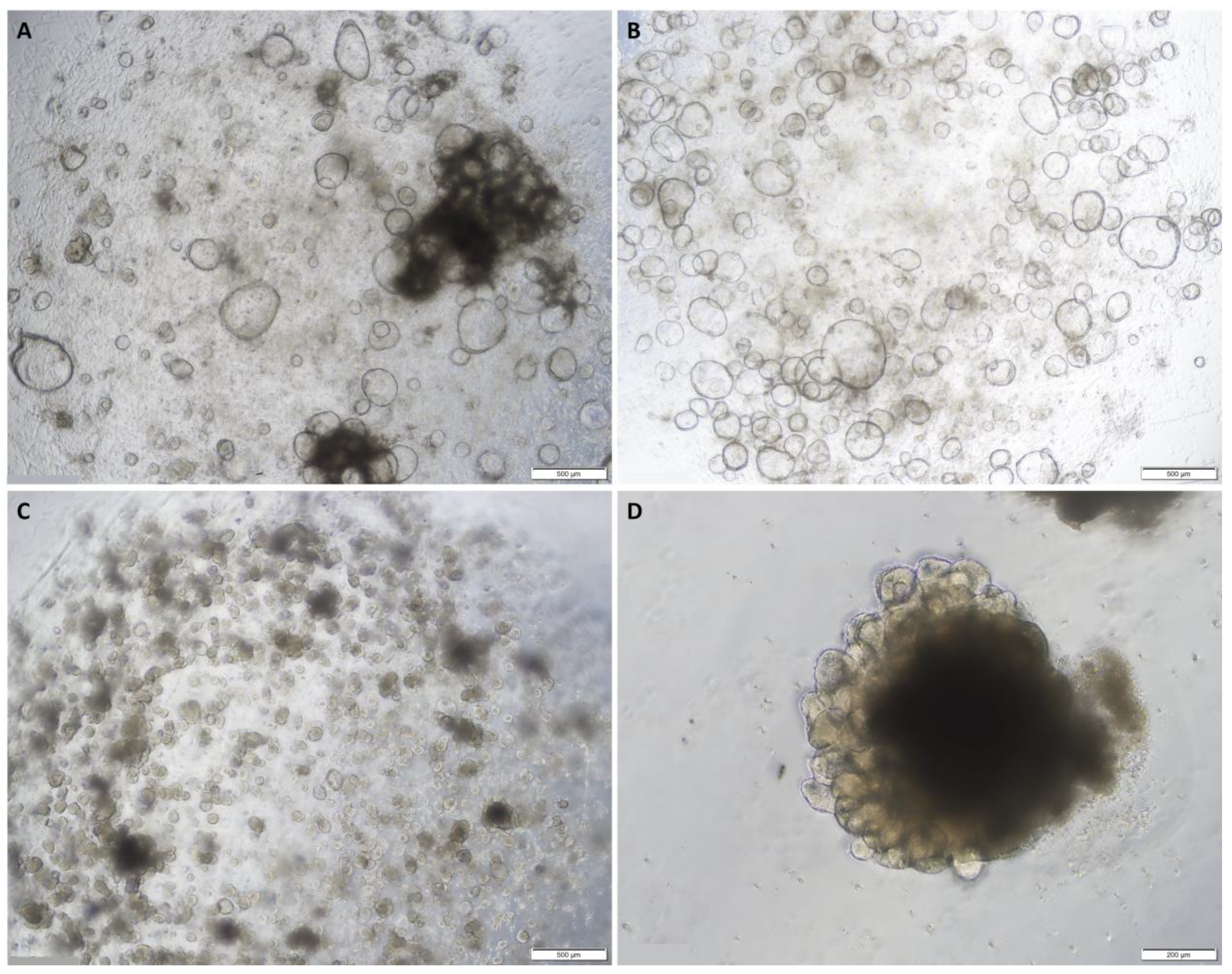This image comprises a quartet of square microscope slides, each labeled A, B, C, and D, arranged in a grid. The backgrounds of all four slides vary from light gray to white, showcasing distinct cellular patterns indicative of different sample conditions. 

Slide A, positioned in the upper left, features a dispersed set of mostly colorless cells outlined in dark shades, such as black or gray, with an annotation of 500 in the lower right corner. The cells appear as small circles spread thinly across the slide. 

In the upper right, Slide B displays a greater concentration of lighter-colored cells with a corresponding label of 500. These cells are marked by a lack of dark patches that are seen in Slide A. 

Slide C, found in the lower left, presents a dense clustering of smaller cells that appear gelatinous, almost reminiscent of a jellyfish. The cells are smaller but more numerous than in the other slides, and the sample retains a 500 annotation.

Finally, Slide D, located in the lower right, is dominated by a concentrated dark patch, possibly indicating a pathological condition like cancer, surrounded by a few individual cells. This slide is distinguished by a 200 annotation. The outer edge of Slide D remains relatively clean, forming a stark contrast with the central dark mass. 

Each slide methodically captures distinct characteristics of cellular formations, providing a comprehensive view of varying sample states.